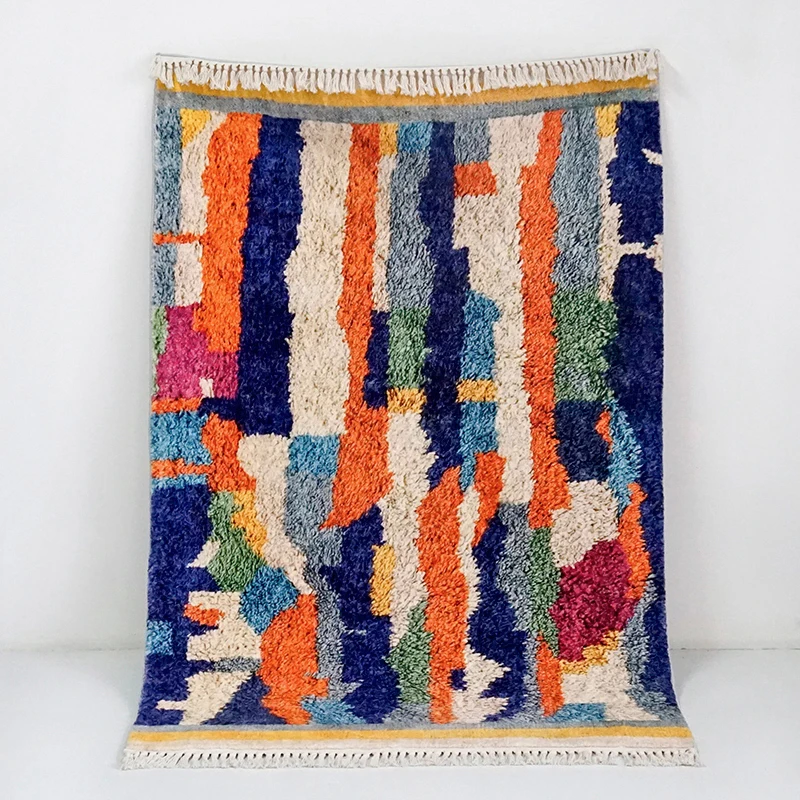The photograph captures a vibrant and textured quilt, hanging against a white background that extends to the floor. The quilt, which could also be seen as a rug or wall hanging, is distinguished by its intricate array of colors and patterns. From the top, white fringes cascade down, followed by a horizontal yellow strip, and then a gray line. The majority of the quilt showcases a shaggy texture adorned with an irregular yet harmonious mix of stripes and shapes in colors such as gray, white, orange, blue, light blue, yellow, and bright pink. Among these are notable irregular shapes, including an orange carrot-shaped triangle and a burgundy blob towards the lower right. Small orange lines extend perpendicularly from the main orange stripes. At the bottom, the pattern concludes with another series of blue and yellow lines, terminating in a neatly arranged white fringe that rests on the floor. The quilt's seemingly random yet captivating arrangement of colors and shapes gives it a whimsical, well-traveled appearance.